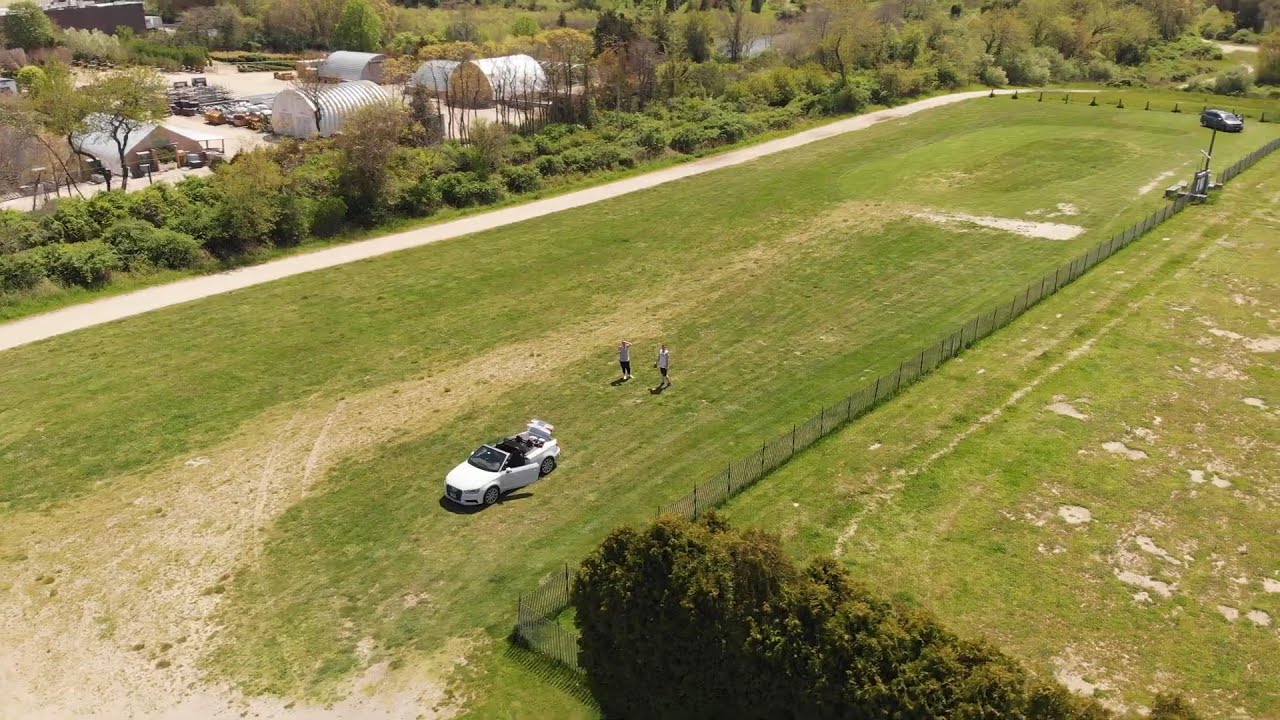The image is a color, landscape-oriented drone photograph taken from a higher vantage point, capturing a zoomed-out view of a large, grassy, oval-shaped field on a sunny day. Dominating the wide section of the field in the bottom left corner is a white convertible car with its driver's side door and trunk lid open. About 15 to 20 feet behind this car, two young men can be seen; one is wearing a white t-shirt and dark shorts, with his arms outstretched, while the other is clad in a grey t-shirt and dark shorts, simply walking. Their shadows stretch out in front of them, indicating that the sun is positioned behind them. There is a chain-link fence running from the bottom right and curving towards the middle and back again towards the top right, connecting to a large shrub. On the other side of the field, a minivan is parked with a couple of people standing near it. The field narrows toward the upper right corner of the image, bordered by a row of shrubs and what appears to be a nursery. The upper left part of the photograph features several greenhouse-type structures surrounded by trees, while a vacant pasture and an overhead light structure are visible in the top right section. The photograph’s representational realism offers a detailed and clear view of the setting, emphasizing the contrasts and elements within the field.